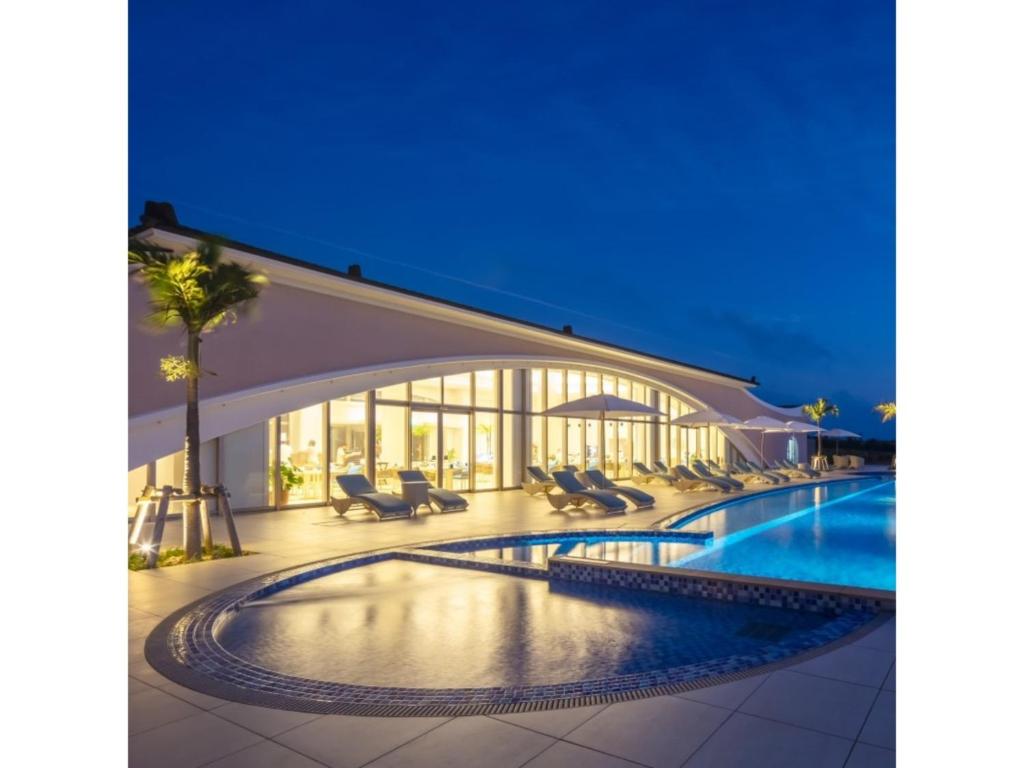The image captures an opulent, likely nighttime, outdoor scene of a luxurious hotel or high-end residence featuring an expansive, uniquely shaped swimming pool. The pool area is adorned with numerous padded deck chairs and umbrellas, positioned for ultimate relaxation. On the left-hand side, a prominent palm tree stands, with additional palms visible towards the back, their silhouettes and reflections enhancing the tranquil ambiance. The large pool is thoughtfully designed with rounded sections and includes a smaller, possibly half-moon-shaped pool adjacent, likely serving as a hot tub or wading area. The surrounding deck is lined with both large square tiles and smaller blue tiles around the pool and hot tub, adding to the aesthetic appeal.

Behind the pool, an impressive building with a distinctive curved façade and panoramic windows emits a warm, inviting yellow light that spills into the night. This structure seems to contain a dining area or restaurant, where a couple of people and tables are visible. The building's archway, stretching almost the entire length of the structure, further accentuates its grandeur. Small patches of grass interspersed within the tiled area provide bases for the palm trees, giving a touch of greenery amidst the architecture. The dark blue, gradient sky, almost devoid of clouds, sets a serene backdrop, suggesting either nighttime or twilight, with one observer noting the possibility of a star or satellite streaking across.

Overall, the scene exudes luxury and relaxation, with illuminated blue pool lights reflecting off the water, enhancing the serene, nighttime atmosphere.